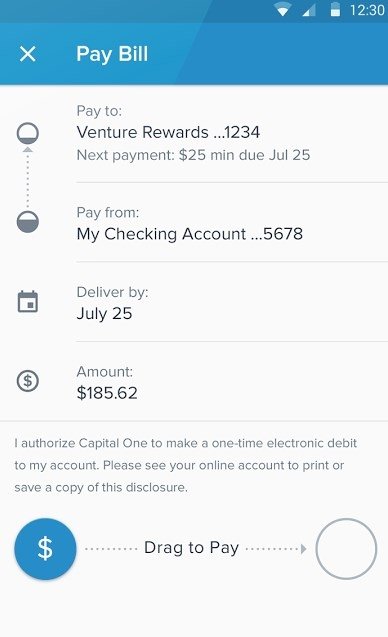**Detailed Caption:**

This image is a detailed screenshot of a BillPay screen within a mobile application.

At the very top of the screen, a header with two shades of blue creates a dynamic design, with a lighter blue on the left transitioning at an angle into a darker blue on the right. Displayed prominently in the top-right corner of the screen are several status icons:
- A halfway-full white Wi-Fi signal symbol.
- To the right of the Wi-Fi symbol, a mobile signal icon that resembles a triangle oriented with its long face up and right, indicating halfway full.
- Next to the mobile signal icon is a vertically positioned battery symbol, half-filled with white.
- Adjacent to the battery icon, the current time, "12:30", is displayed in white text.

On the bottom-left side of the blue header, there's a white "X" icon intended for users to exit or close the screen. To the right of the "X" icon, the text "PayBill" is shown, indicating the function of the screen.

The main portion of the page, beneath the header, features a light gray background with several rows, each dedicated to different payment details, identifiable by their distinct icons and separated by thin lines:

1. **First Row:**
   - Icon: A gray-outlined circle, partially filled with gray at the bottom.
   - Label: "PayTo"
   - Details: "Venture Rewards...1234"
   - Next Payment Due: "$25"
   - Minimum Due: "July 25"

2. **Second Row:**
   - Icon: Similar to the first, but filled about two-thirds with gray, accompanied by a dotted arrow pointing up to the first circle.
   - Label: "PayFrom"
   - Details: "MyCheckingAccount...5678"

3. **Third Row:**
   - Icon: A calendar
   - Label: "Deliver by"
   - Details: "July 25"

4. **Fourth Row:**
   - Icon: A dollar sign inside a gray circle
   - Label: "Amount"
   - Details: "$185.62"

Below these rows, a disclaimer reads: "I authorize Capital One to make a one-time electronic debit to my account. Please see your online account to print or save a copy of this disclosure."

At the very bottom of the screen, instructions are provided for completing the payment: "Drag to Pay", accompanied by a user interface feature with two circles. The first circle on the left contains a dollar sign, and arrows point from it to an empty gray circle on the right, indicating the drag action needed to complete the payment process.